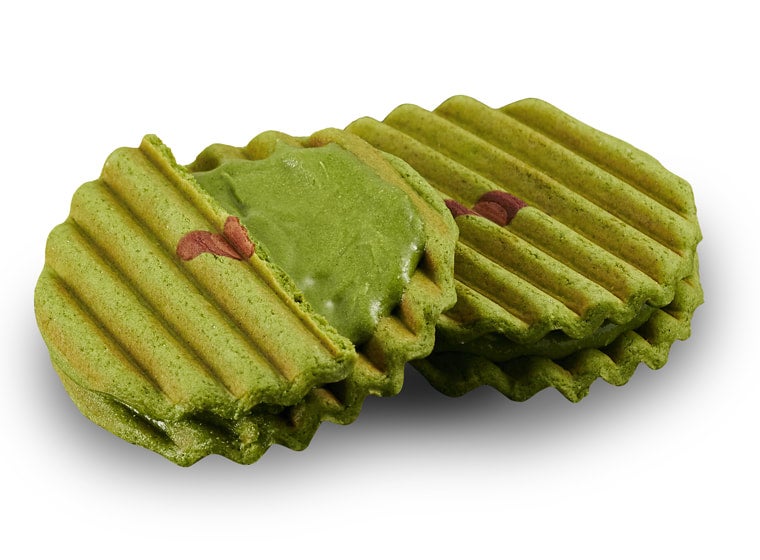The image features a pair of green, wafer-like objects that resemble cookies or biscuits. Each piece has distinct ruffled or crinkle-cut edges reminiscent of a ruffled potato chip, but softer in texture. The objects appear to be green with a slimy or fluid-like center and a few red stains or specks on the surface, possibly indicating some spice or seasoning. One of the cookies is leaning on the other, and the one on the left has a portion of its top layer broken away, providing a clear view of its green, almost sauce-like interior. The outer surface has a mix of dark green shades with occasional white speckles, and the entire scene is set against a stark white background. The overall appearance suggests they may be a type of baked or molded food item, with a curious combination of solid and slimy textures.